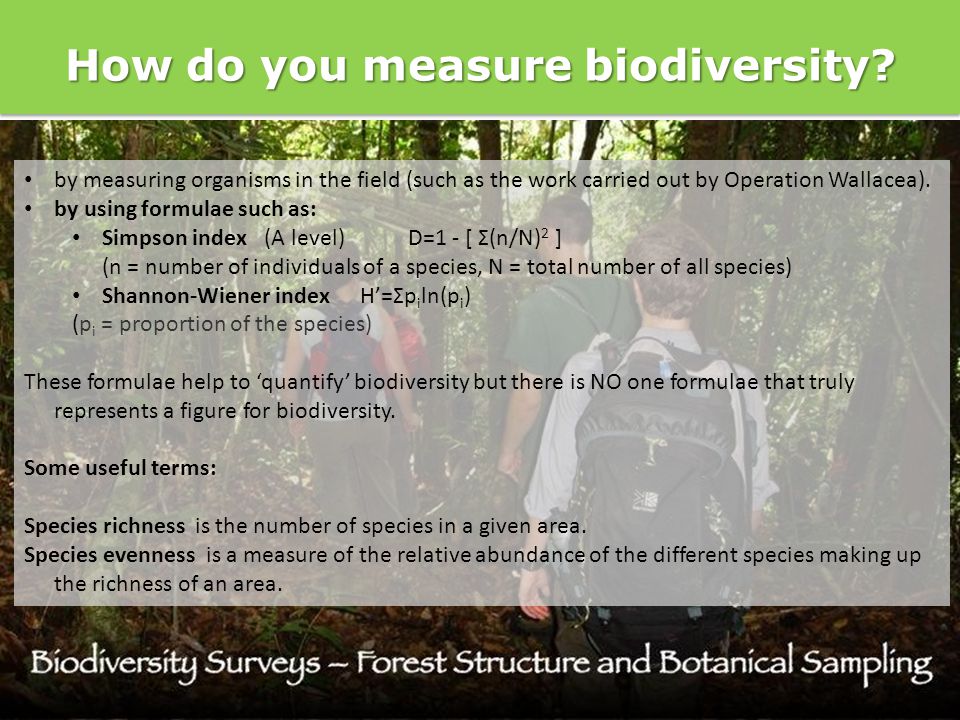The image is of an informational page or PowerPoint presentation slide created on a computer, designed to detail how to measure biodiversity. At the very top, there's a green rectangular banner with white block lettering that reads, "How do you measure biodiversity?" Below this banner, there's a thin white strip separating it from the main content. The main background image is a natural scene showing people hiking through a forest, with trees and foliage subtly visible. The hikers are only seen from the back, featuring details such as their backpacks and clothing. Foremost in the image is an individual with short brown hair, wearing a gray button-up shirt and a black backpack; others have varying outfits including green and whitish-gray shirts, and backbacks in black and red hues.

Superimposed over this forest scene is a light gray rectangular cutout with black text. The text includes:

- Bullet points explaining methods for measuring biodiversity, such as field work by Operation Wallacea.
- Formulas detailing the Simpson Index and Shannon-Wiener Index for quantifying biodiversity.
- Explanations that no single formula can fully encapsulate biodiversity.

At the bottom of the gray box, there's a section titled "Some useful terms," defining key concepts:
- "Species richness" is noted as the number of species in a given area.
- "Species evenness" is defined as the measure of the relative abundance of different species making up the richness of an area.

In the background at the bottom, in a stylized white font, it reads: "Biodiversity surveys – forest structure and botanical sampling."